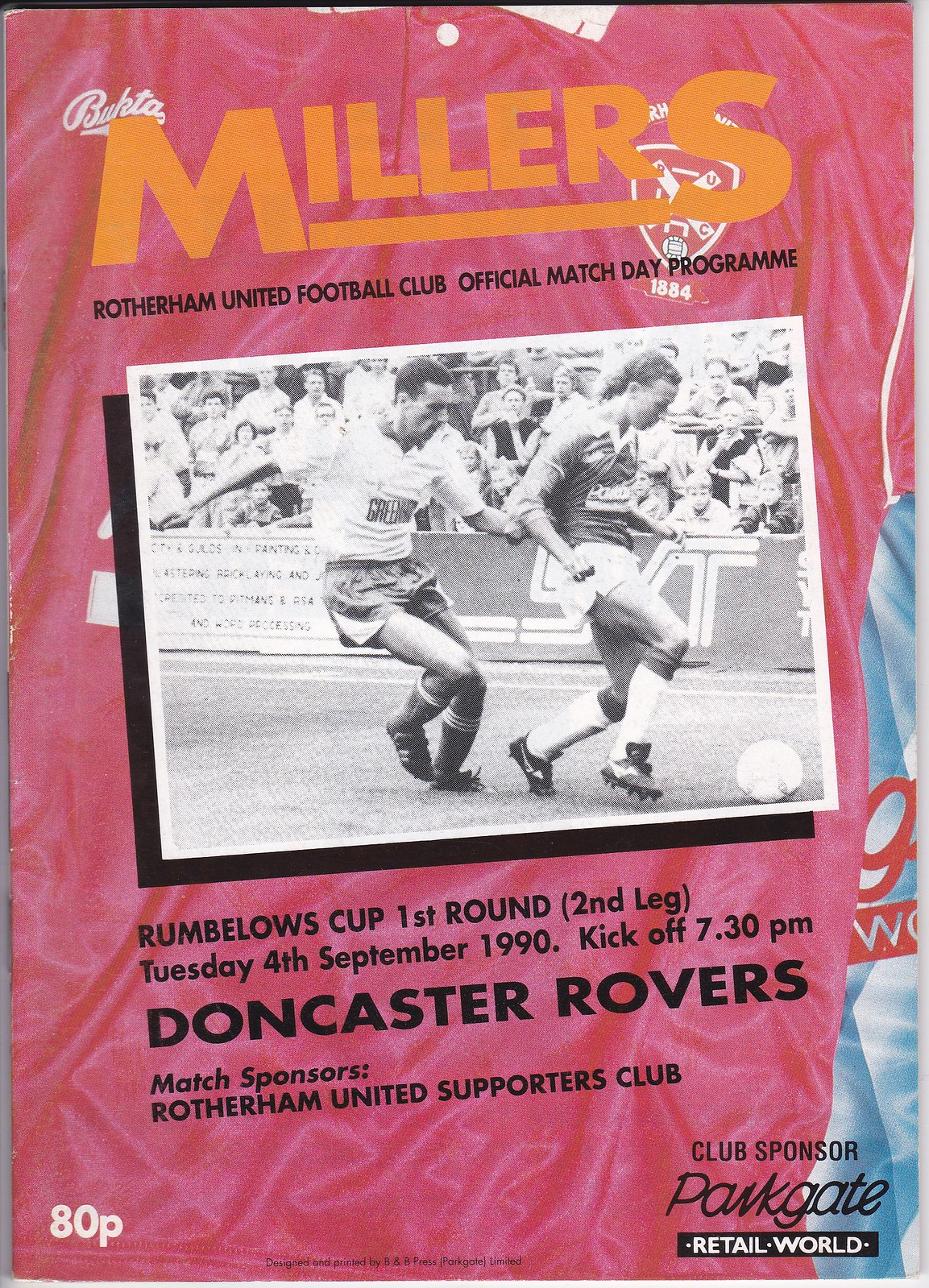This is a program for a soccer team, primarily in shades between hot pink and purple, with an orange header that reads "Millers." Beneath the header, in tiny black print, it says "Rotherham United Football Club Official Match Day Program." The cover displays a textured, rumpled tablecloth-like backdrop with blue and red elements on one side, hinting at additional graphics. Below the title is an insignia resembling a shield.

The main feature is a black and white photograph of two players—one in a white shirt and the other in a dark shirt—caught in action with their knees bent, heels off the ground, and a soccer ball between them, while spectators watch from the bleachers. The program is for the Rumbelows Cup, First Round, Second Leg, held on Tuesday, 4th September 1990, with kickoff at 7:30 p.m., against Doncaster Rovers. Match sponsors are the Rotherham United Supporters Club and Parkgate Retail World, noted near the bottom. The price, indicating "ADP," is located at the bottom left corner.